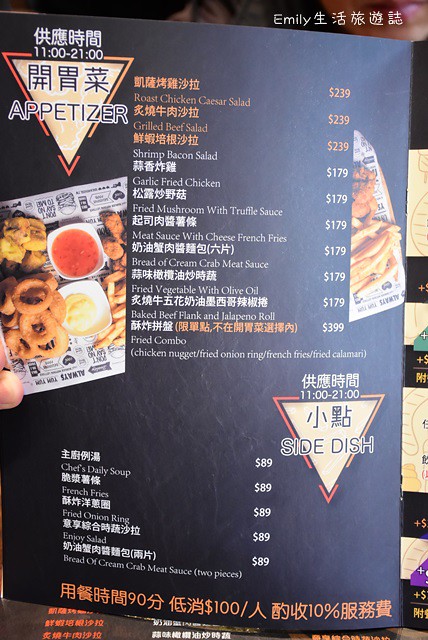In the image, a black menu is displayed upright, featuring both a foreign language and English translations beneath each item. The menu showcases colorful photographs of various dishes including onion rings, red sauce, cream-colored sauce, and French fries. The listed items from top to bottom are as follows: Roast Chicken Caesar Salad, Grilled Beef Salad, Shrimp Bacon Salad, Garlic Fried Chicken, Fried Mushroom with Truffle Sauce, Meat Sauce with Cheese French Fries, Bread with Cream Crab Meat Sauce, Fried Vegetables with Olive Oil, Flaked Beef Flank and Jalapeno Roll, and a Fried Combo. The Fried Combo includes chicken nuggets, fried onion rings, French fries, and fried calamari. A section marked with a downward-pointing triangle labeled "Side Dish" is also visible, along with a repeated price of $89.89 in colored numbers, creating some confusion about the pricing.